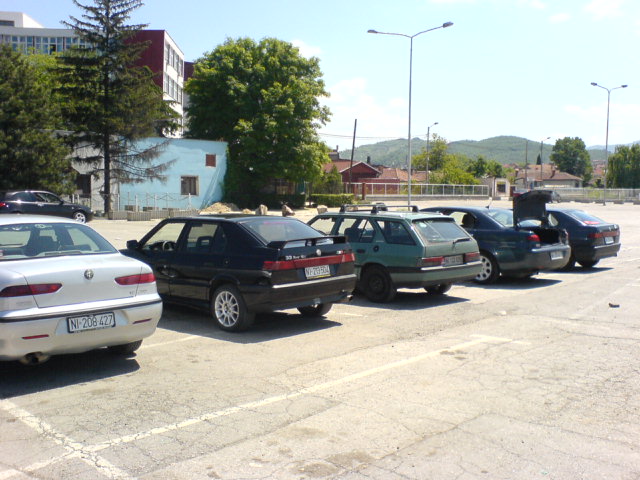The photograph captures a bright, sunny day in a gray, tarmac-covered parking lot, featuring five cars parked in a row, each demarcated by white parking lines. The cars, from left to right, include an off-white vehicle, a black car, an older medium green wagon, a dark blue car with its trunk wide open, and another dark blue car with its trunk closed. The license plate of the leftmost car, clearly visible, reads NI208427. In the background, a series of buildings can be seen, including a multi-storied red and white building with numerous windows, and another building that is white on the left and light blue on the right. A tall, dark green tree stands in front of the white building. Further back, hills covered in greenery are visible beneath a blue sky streaked with a few white clouds. Additionally, there is a black car parked horizontally in the distance, further emphasizing the structured layout of the scene. Overhead lights dot the parking lot, presently off, contributing to the overall organized and serene atmosphere of the photograph.